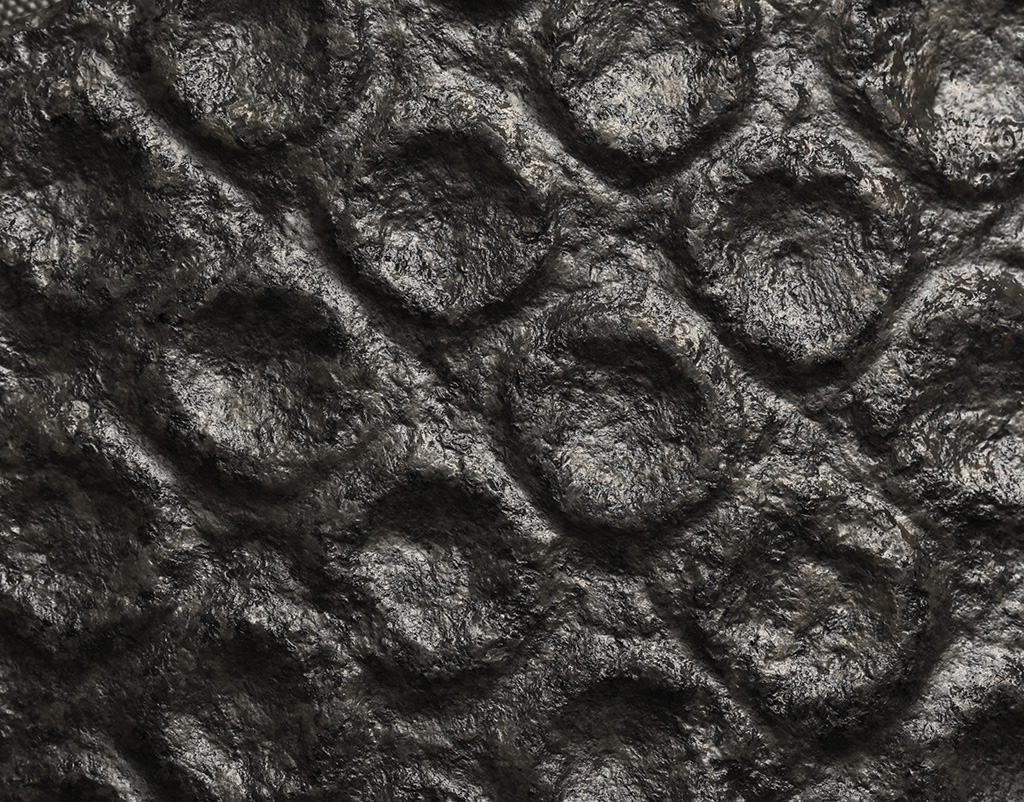The image depicts a detailed pattern composed of blacks, grays, and highlighted whites, resembling a wall or rock formation with numerous divots and crater-like structures. The light source is emanating from the upper right-hand corner, casting diagonal shadows across the surface. The pattern features rectangular shapes, each housing a raised, circular area that looks like a crater. This textured surface appears to have grooves running diagonally and vertically across it, giving the impression of animal skin or eroded material, possibly an old or historic wall often seen in museums. The material's surface texture evokes a sense of aged stone or mud, adding to the impression of antiquity and distinct character.